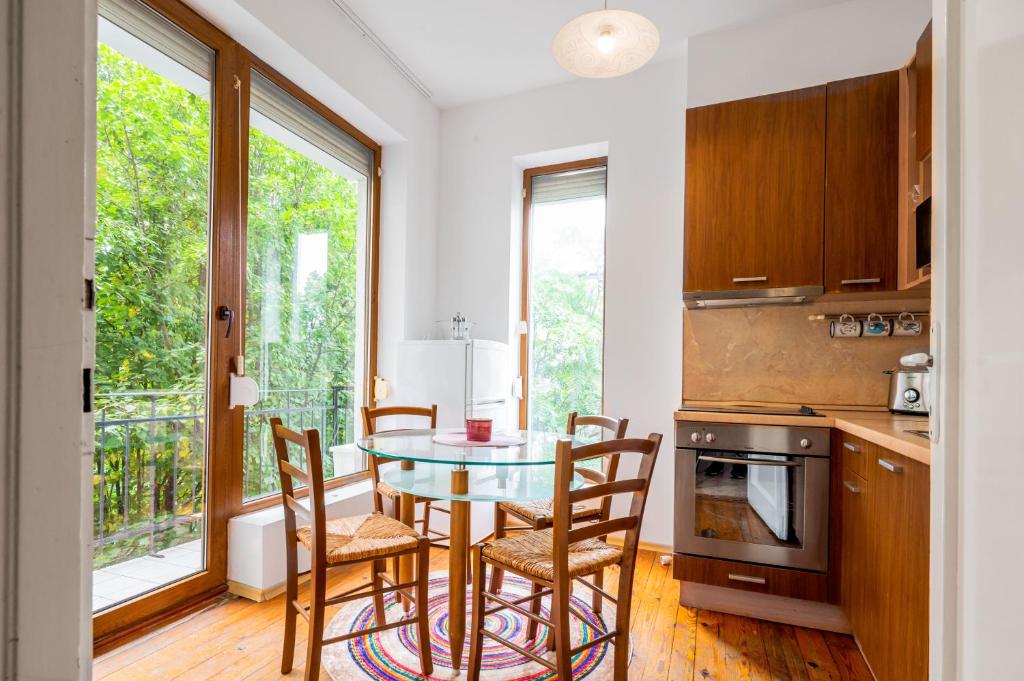The image depicts a small, staged kitchen area within a cozy apartment or cabin, illuminated by a blend of natural and artificial light. The central focus is a small glass-top dining table with four chairs, featuring wooden frames and wicker seats, all positioned on a circular rug. Brightly colored wooden cabinets line the back wall, framing a countertop that might be stone, adorned with a silver oven and a toaster. A compact, white refrigerator fits snugly between two windows in one corner. The room boasts ample light from a large window and a glass French door with a black handle that opens out to a balcony, revealing trees outside. Additional details include some coffee cups hanging and a glass door in the center of the kitchen area. There are no people or text present in the image.